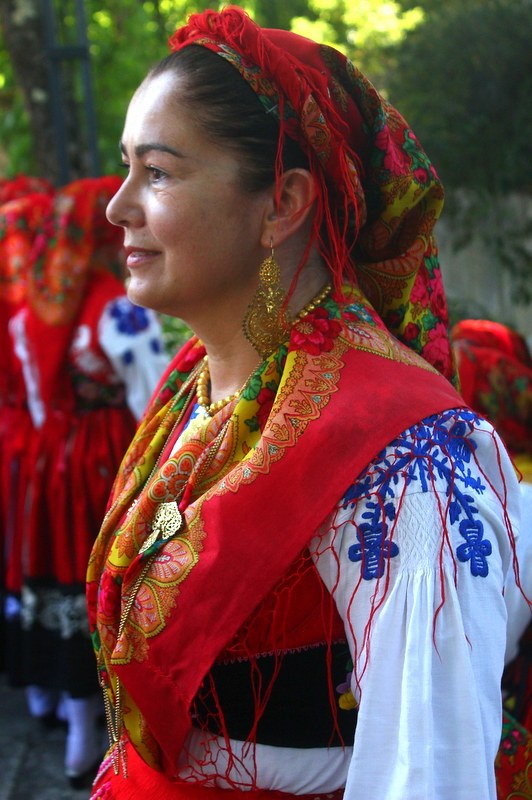In this outdoor, daytime photograph set in a wooded park, we see a side profile of a Caucasian woman, likely in her 40s, adorned in traditional Eastern European folk attire. Her black hair is styled under a red, floral headdress. Ornamenting her look are large golden earrings and a matching gold necklace. She gazes away from the camera, adding a contemplative tone to the image.

Her ensemble features a white shirt embroidered with blue flowers and red designs, complemented by a black vest. Draped over her shoulders is a vibrant red scarf adorned with orange floral patterns. In addition, a black cummerbund accentuates her waist.

In the blurred background, another woman is seen wearing a similar outfit, comprising a red skirt, a red vest, and a white shirt with blue floral embroidery, all set against a backdrop of trees illuminated by the sun. The detailed ethnic attire of both women is a vivid representation of their cultural heritage.